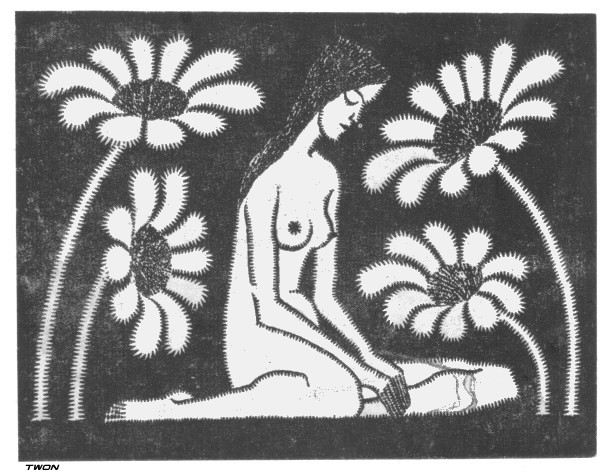This black-and-white painting, signed by T-W-O-N, portrays a naked woman with black hair sitting in a field of oversized sunflowers. The woman, who appears either sad or pensive, is depicted looking down at her hands, which are held closely together but not entwined. She is sitting on the ground, seemingly immersed in her thoughts. The striking sunflowers, almost as tall as the woman, are characterized by their long stems, black centers, and about ten white petals each. These flowers, reminiscent of the 1960s hippie era, seem to lean towards her, almost as if offering protection or comfort. The entire scene, set against a stark black background, is rendered in a style with solid colors and lines, devoid of shading, reinforcing the somber and reflective mood of the image.